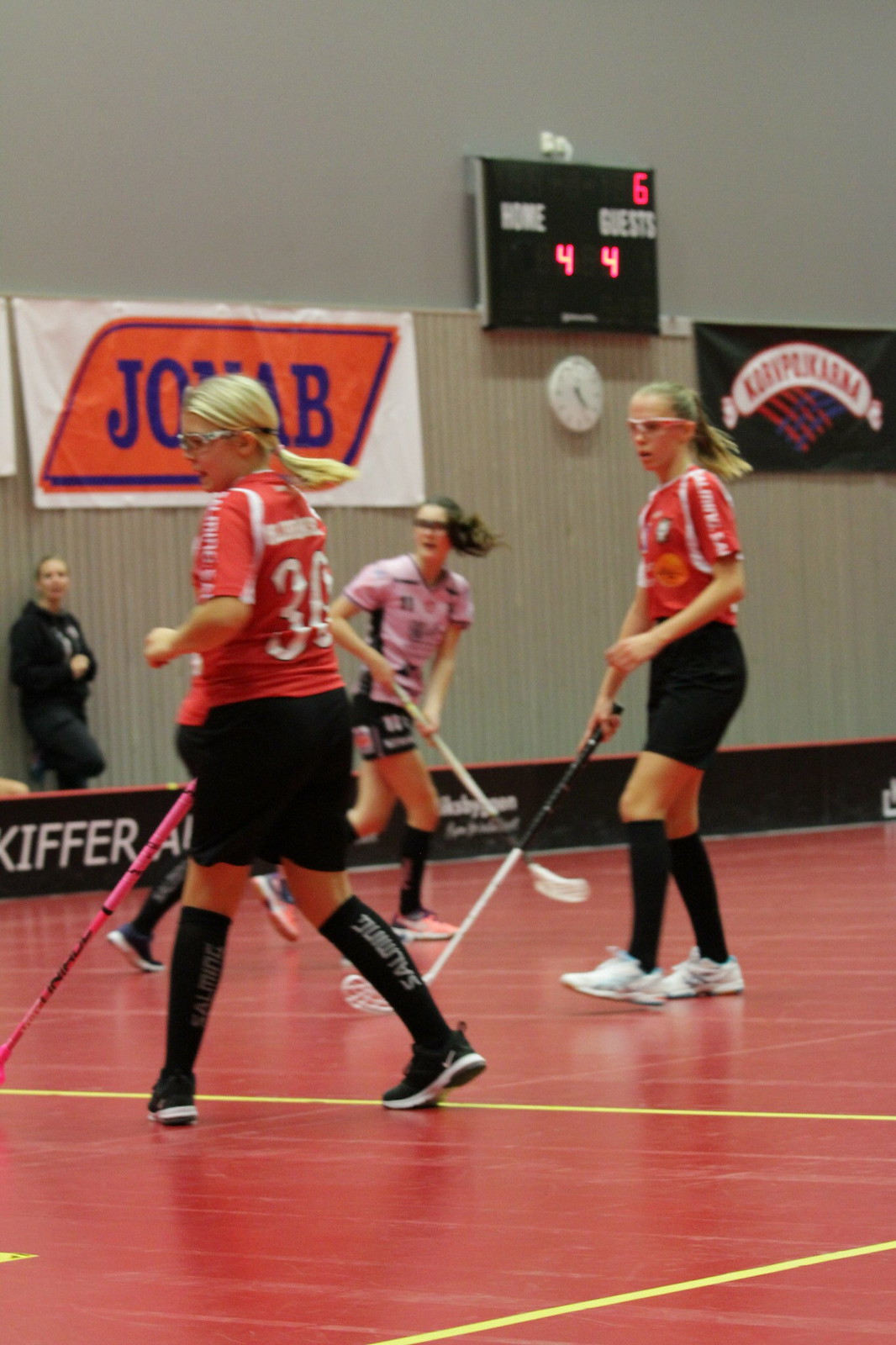The photograph captures an intense moment in an indoor hockey game inside a gymnasium with red flooring marked by yellow lines. The scene is dominated by three girls in the foreground, all focused towards the left with their hockey sticks poised for action. Two of the girls are dressed in red, white, and black uniforms, while a third girl, positioned between them, wears a pink and black uniform. The score, displayed on a grey scoreboard mounted on the back wall, reads Home: 4, Guest: 4, with a noticeable '6' in the upper right corner. Below the scoreboard, a white round clock can be seen. Flanking the clock are two banners, one partially obscured but reading "JONAB" in blue text on an orange block, and the other a black banner with indistinct text. Additional players are visible in the background, with a few girls off to the side watching the game. The detailed background elements, including the scoreboard, clock, and banners, add depth and context to this dynamic sports scene.